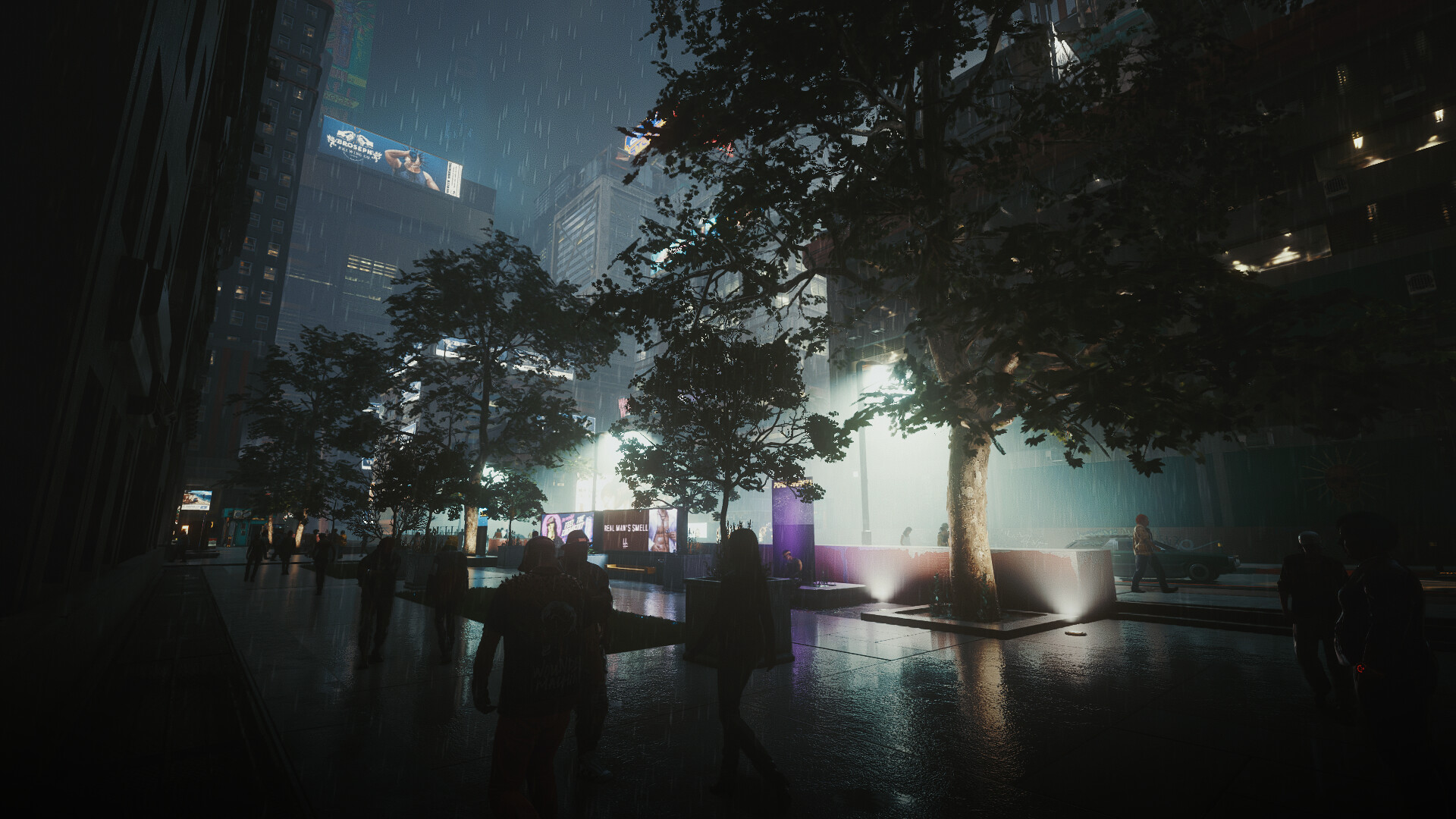This cinematic nighttime scene, potentially a computer-generated rendering or a video game screenshot, captures a vibrant cityscape with striking realism. At the heart of the image is a bustling pedestrian walkway bordered by towering buildings on either side. A row of trees lines the path, illuminated from below by strategically placed ground lights that cast an ethereal glow on both the foliage and the wet pavement. The silhouettes of numerous pedestrians can be seen moving along the walkway, bathed in shadow and adding life to the scene. Above, a persistent rain showers down, creating a reflective, slick surface on the ground and contributing to the cold, atmospheric mood of the image.